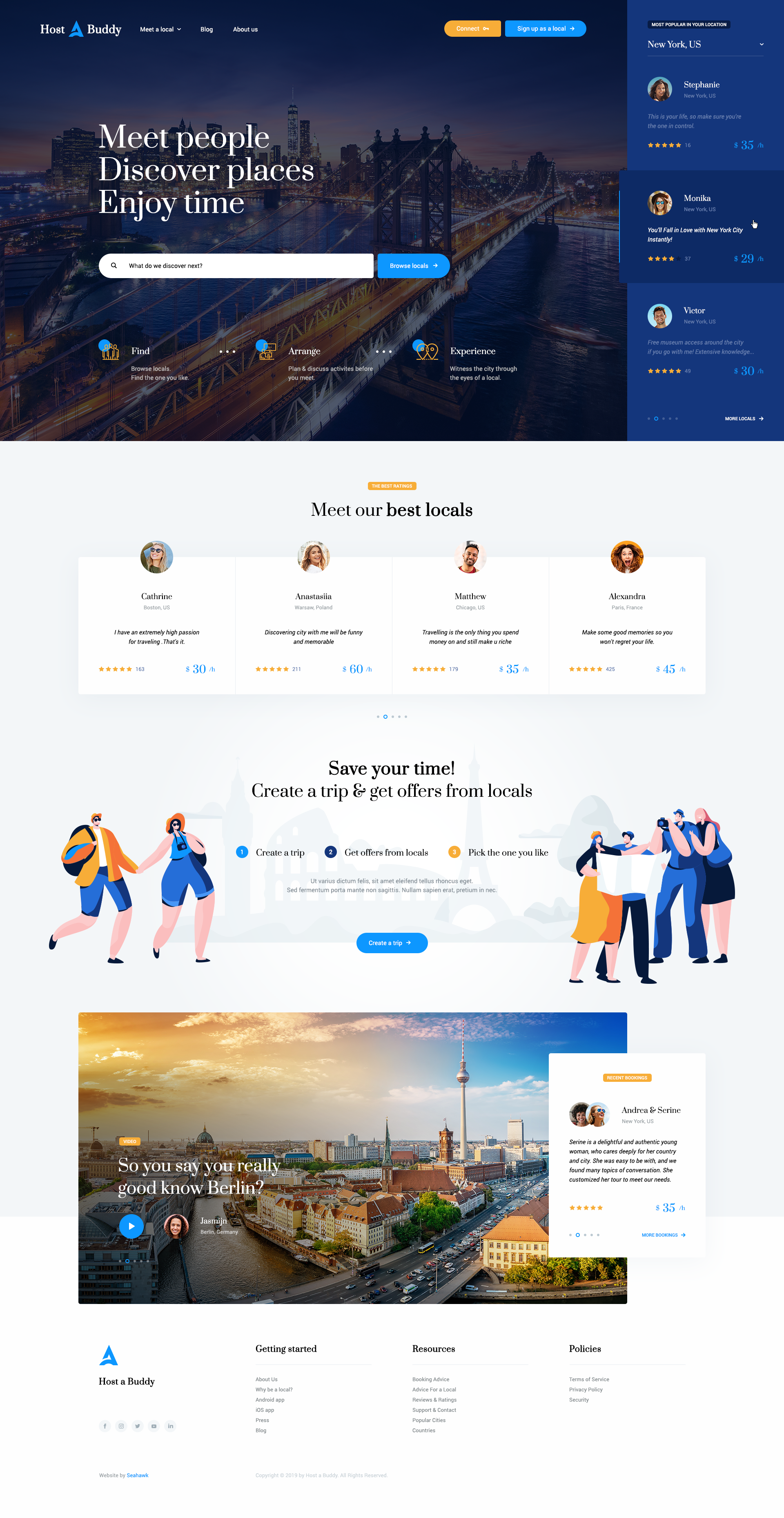**Detailed Caption for "Host a Buddy" Travel Web Page Screenshot**

This screenshot captures the home page of "Host a Buddy," a travel platform designed to connect travelers with local guides. The main banner, set against a stunning nighttime cityscape featuring a bridge, prominently displays the text "Meet People, Discover Places, Enjoy Time." Below this banner is a search bar encouraging users to explore with the prompt, "What do we discover next?"

The page is divided into several organized sections. The first four sections are titled: "Find," "Arrange," "Experience," and "Meet Our Best Locals." These sections guide users through the process of finding and arranging their travel experiences.

In the "Meet Our Best Locals" segment, there are profiles of four standout local guides:
1. **Catherine, Boston, USA:** "I have an extremely high passion for traveling."
2. **Anastasia, Warsaw, Poland:** "Discovering each city with me will be funny and memorable."
3. **Matthew, Chicago, USA:** "Traveling is the only thing you spend money on that will make you richer."
4. **Alexandra, Paris, France:** "Make some good memories so you won't regret your life."

Each profile features a small round picture of the guide, their name, location, a brief personal description, a star rating, and an hourly rate.

Adjacent to this is a section emphasizing the ease and efficiency of the platform: "Save your time, create a trip, and get offers from locals."

A highlighted feature location showcases Berlin, Germany along with a scenic image portraying the city's skyline. The site also includes a recently booked guide profile for Andrea and Serene in New York. Their description reads: "Delighted and authentic young woman who cares deeply about her country and its city. She was easy to relate to, found many topics of conversation, and customized her tour to meet our needs."

The navigation bar at the top provides links to various parts of the website, while the footer offers connections to additional resources and policy information.